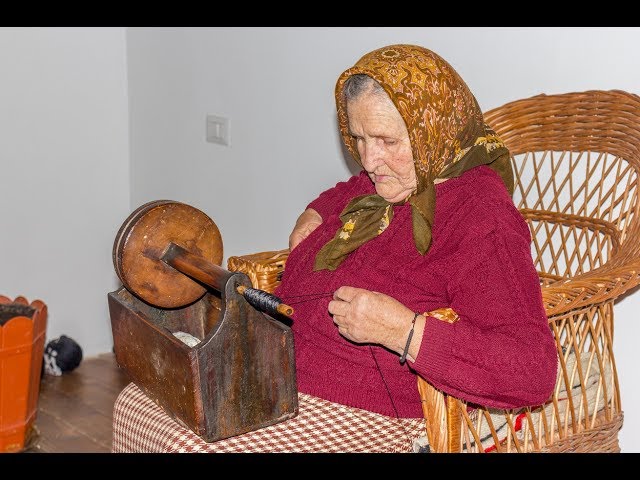The photograph features an elderly woman, likely in her 80s, seated in a high-backed wicker chair which almost engulfs her slight frame. She has gray hair partially covered by a brown kerchief adorned with earthy, paisley patterns, commonly referred to as a babushka. Dressed in a burgundy shirt and a plaid skirt, she is meticulously manipulating thread on what appears to be a manual sewing machine or an old-fashioned spinning device. The apparatus resembles a rectangular-shaped bucket with a spindle mounted on top, around which the thread is coiled. She is pulling the thread with her left hand, her expression one of concentration. The scene is set in a modest, white-walled room with a wooden floor, where scattered objects and a light switch can be seen in the background, lending a homely, slightly cluttered atmosphere to the setting.